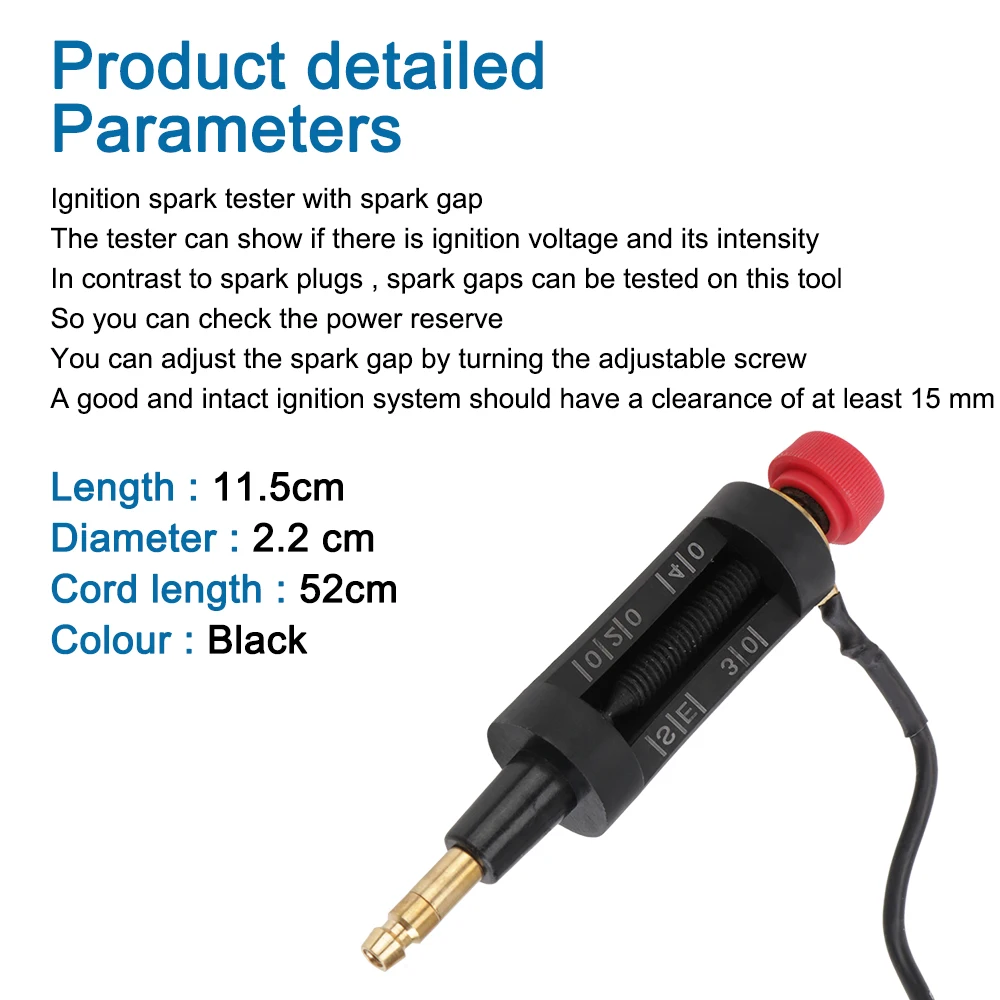This image showcases a detailed advertisement for an ignition spark tester with spark gap functionality. At the top, large blue text indicates "Product Detailed Parameters." The tester, primarily black in color, features a distinct bright red adjustable screw cap for modifying the spark gap. The product is designed to demonstrate the presence of ignition voltage and its intensity compared to traditional spark plugs, allowing users to check the power reserve of their ignition system. It emphasizes that a well-functioning system should exhibit a clearance of at least 15 millimeters. The image details the dimensions of the device: a length of 11.5 centimeters, a diameter of 2.2 centimeters, and a cord length of 52 centimeters. The tester incorporates a golden plug and a hose attachment, enhancing its functionality. Overall, this tool provides comprehensive measurements and adjustments essential for testing spark gaps effectively.